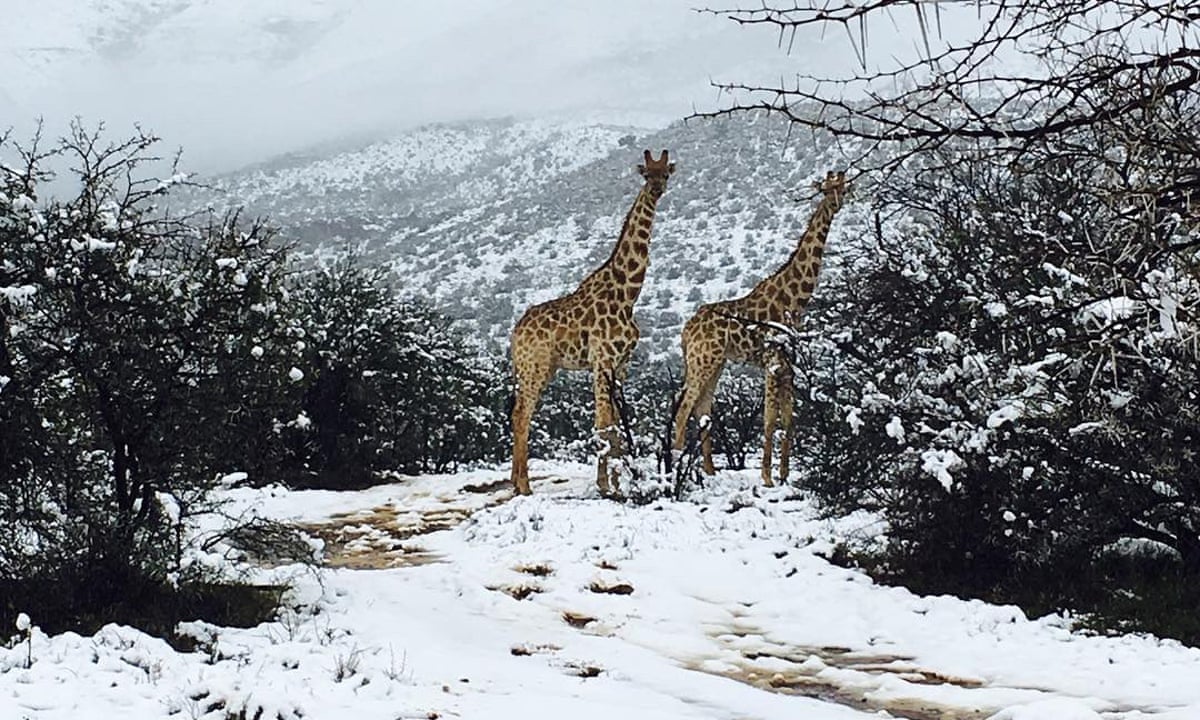In this captivating winter scene, two young giraffes stand side by side, seemingly out of place in their snowy surroundings. Both giraffes are facing right, with one slightly off-center, yet they have turned their heads to look directly at the viewer. The ground and trees around them are blanketed in snow, the tree branches mostly devoid of leaves or covered in blackened snow.

A winding path, starting from the bottom right of the image, curves gently through brambly shrubs and dark, wiry bushes towards the center, leading right to where the giraffes are standing. The ground and distant hills are also covered in a thick layer of snow, adding to the stark and quiet beauty of the scene. The background is dominated by a partially obscured mountain, its peak hidden by low-hanging clouds, which creates a mysterious and serene atmosphere. The juxtaposition of the giraffes in this winter wonderland highlights their misplaced presence, creating a striking and memorable image.